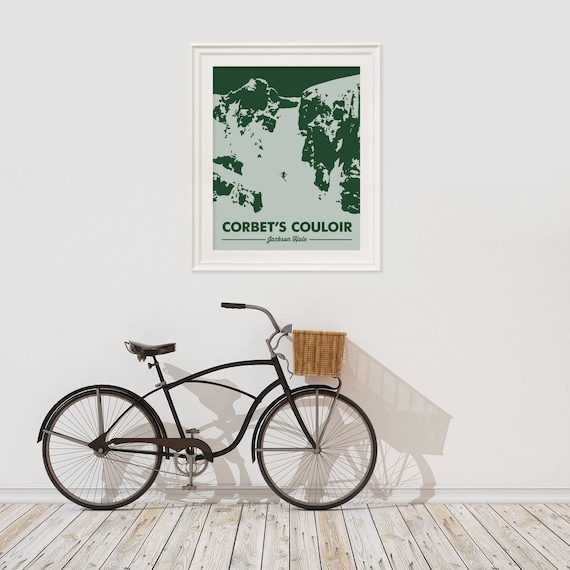In a warmly lit room, illuminated from the upper left, a vintage bicycle is delicately positioned against an off-white wall. The bike, finished in a deep, dark brown hue, features wide, upward-sloping handlebars and a charming light to medium brown wicker basket attached to the front. Resting on light-colored, whitewashed wooden beam floors, the bicycle casts subtle, elongated shadows adding depth to the scene.

Above the bicycle, a vertically oriented rectangular picture frame is mounted on the wall. This frame, crafted from thick, white wood, encloses a monochromatic, slightly retouched image of a mountainous terrain. The peaks and ridges of these mountains are rendered in shades of light gray and dark green, with a lone skier descending the slope towards the lower right corner. Below this outlined depiction, the words "Corbett's Couloir" are inscribed, an homage to the famous ski run in Jackson Hole, Wyoming. The artwork exudes a rustic charm, complementing the nostalgic feel of the scene.